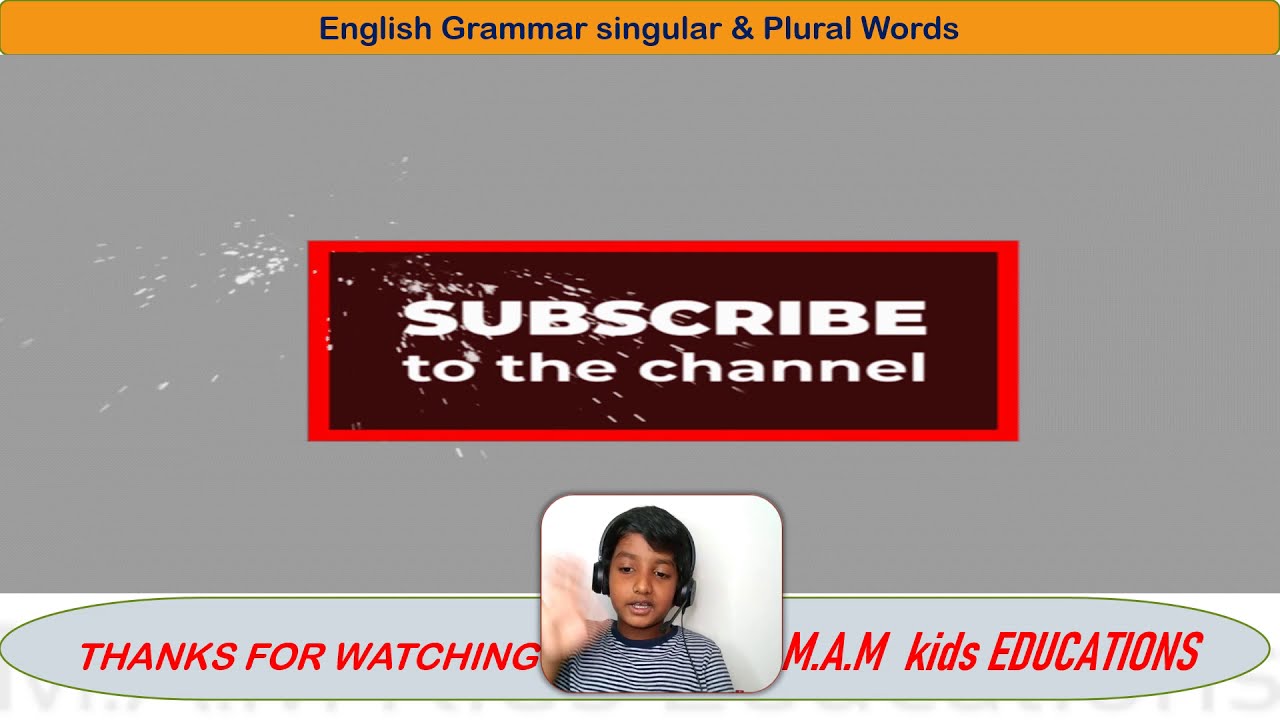The image resembles a frame from a video, featuring a YouTube channel layout where a young boy is presenting educational content. At the top of the image, there is an orange banner with black text that reads "English Grammar: Singular and Plural Words." Below this banner, the background transitions to a large gray area, slightly textured with white splatters.

Dominating the center of this gray background is a gray rectangle with a highlighted red border and a darker red center. Inside this rectangle, in bold white text, it says, "Subscribe to the channel." The text appears centered and is partly obscured by the white splatters on its left side.

Beneath this subscribe content, there is a webcam view of a dark-skinned boy wearing a striped blue shirt and a headset. The boy appears to be waving, indicated by the slight blurriness of his hand. Below his image, there is a light blue speech bubble containing red text that reads, "Thanks for watching. Kids Education." The overall design gives the impression of an amateur yet earnest attempt at creating engaging educational content for viewers.